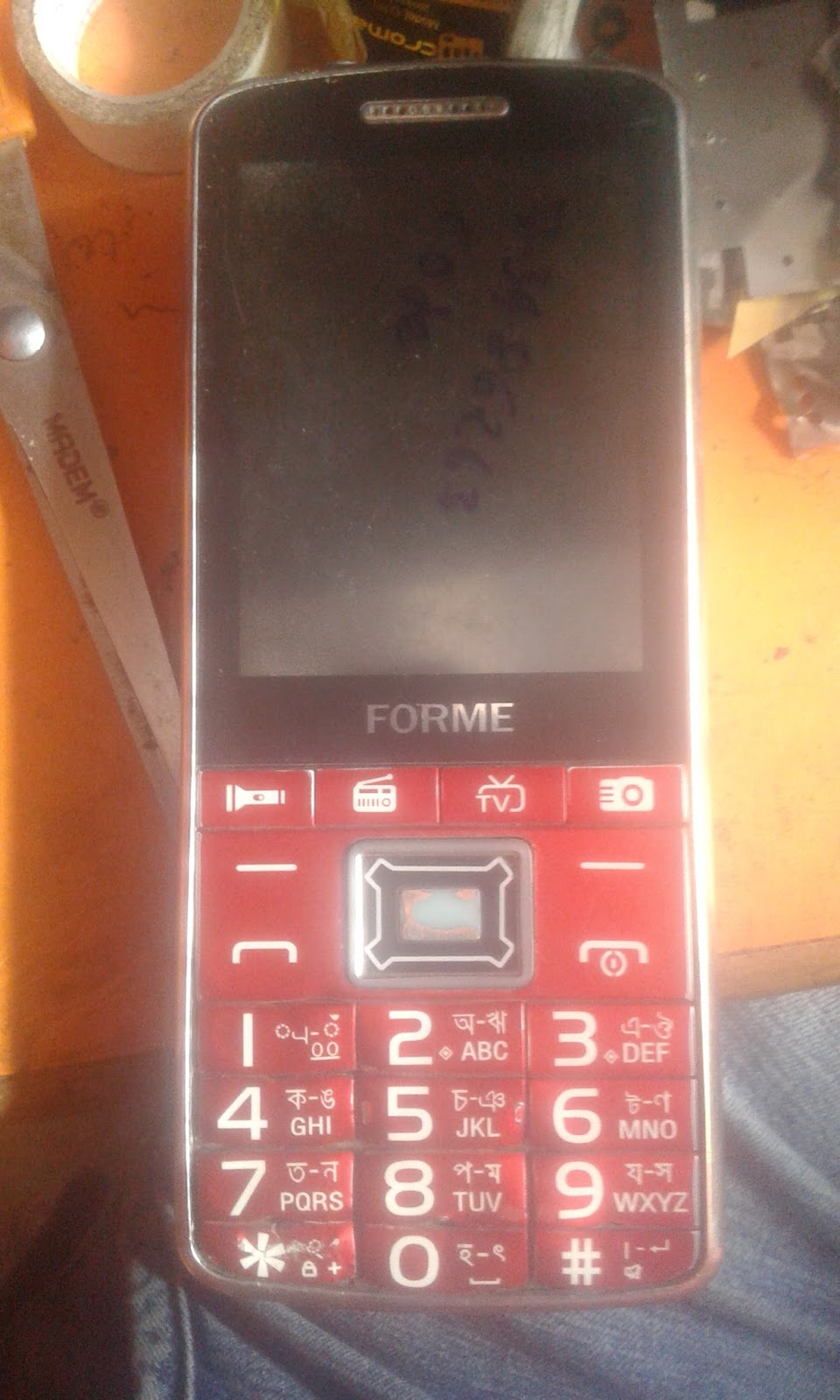The photograph captures a detailed close-up of a rudimentary, old-style cell phone branded "Forme," prominently spelled out in silver letters on a black frame around the screen, which is turned off. The phone is not a flip model but reminiscent of that era, featuring a compact design. The keypad, primarily red with large buttons, dominates the lower two-thirds of the phone. The number pad features standard digits (1-9, 0, *, and #) in white, intersected by English and possibly Korean text. Above the number pad, a large power button sits centrally, flanked by four specialized buttons with icons for a flashlight, radio, TV, and camera. The upper part of the phone maintains a black and silver color scheme, contrasting with the vibrant red of the keypad. The setting includes the phone resting on an orange table, partly covered by what appears to be a pair of silver metal scissors with an orange handle and a roll of clear packaging tape. The image also hints at the presence of blue jeans, possibly indicating human activity nearby, contributing to the photograph's incidental background context.